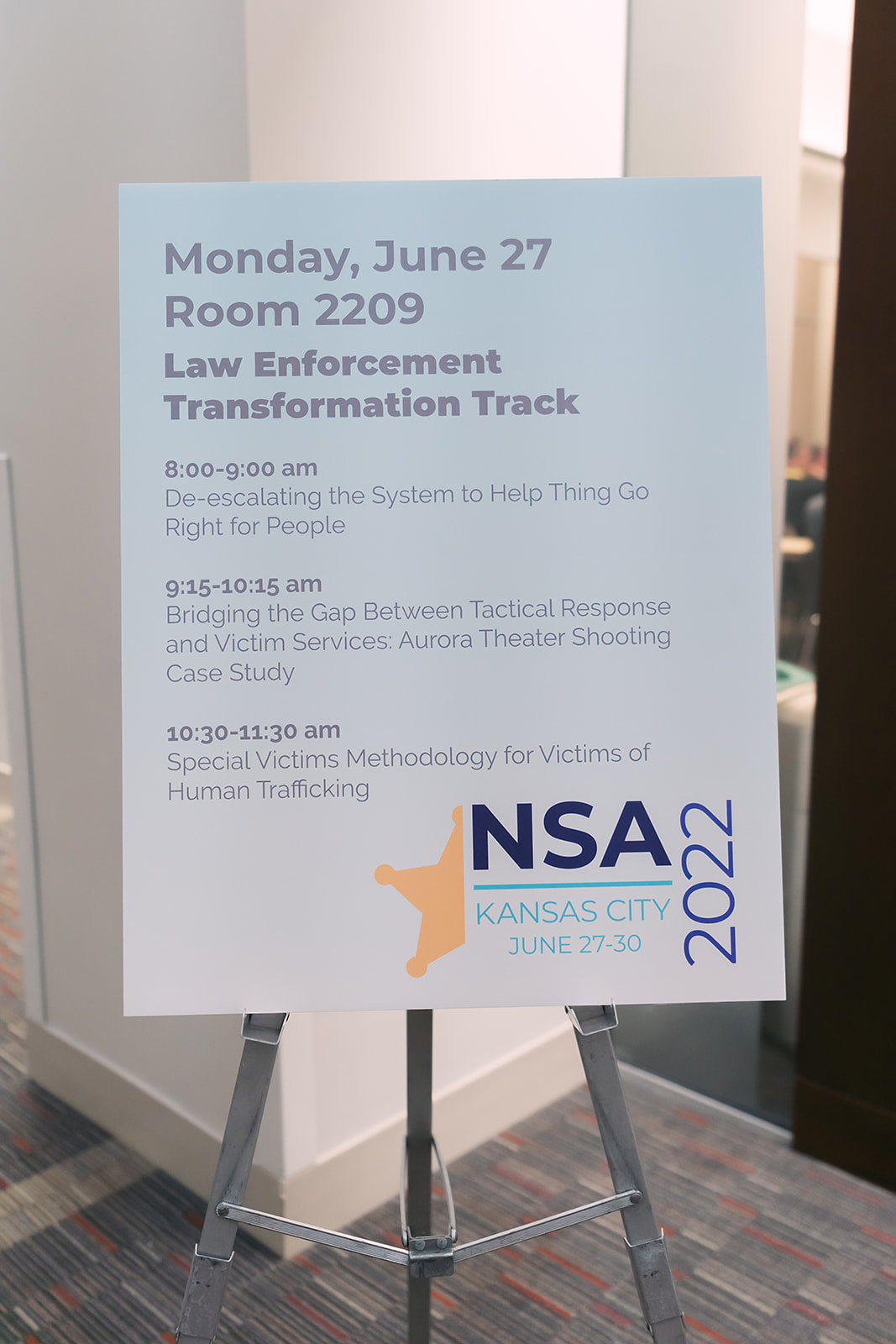The image captures a detailed poster displayed on a grey easel in what appears to be a hotel conference room. The poster, with a light grey background, advertises the "Law Enforcement Transformation Track" happening on Monday, June 27th in room 2209. This track is part of a larger conference, identified by the logo in the bottom right corner that reads "NSA, Kansas City, June 27-30, 2022," beneath a sheriff's badge image. The agenda listed includes: from 8:00 to 9:00 AM, "De-escalating the System to Help Things Go Right for People"; from 9:15 to 10:15 AM, "Bridging the Gap Between Tactical Response and Victim Services: Aurora Theater Shooting Case Study"; and from 10:30 to 11:30 AM, "Special Victims Methodology for Victims of Human Trafficking." The background visible behind the easel features multicolored carpet, and the room itself bears the typical decor one might expect in a hotel's conference space, including white walls and an absence of people.